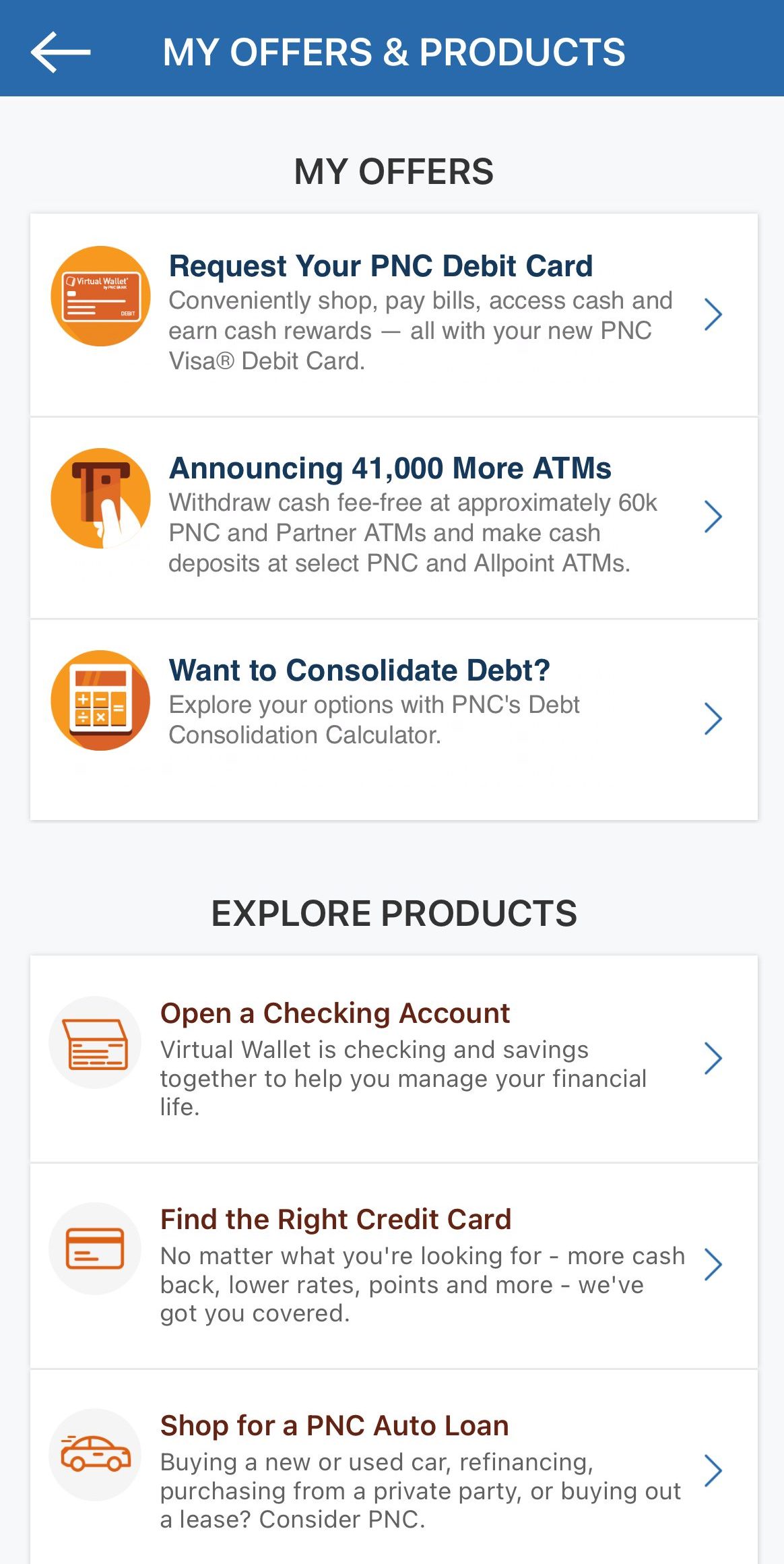Screenshot of the PNC online portal displaying various offers and products. The image highlights several key details:

- "Request your PNC debit card": Easily shop, pay bills, access cash, and earn cash rewards with the new PNC Visa debit card.
- Announcement: Access over 41,000 additional ATMs, making a total of approximately 60,000 PNC and partner ATMs where you can withdraw cash fee-free. Make cash deposits at select PNC and Allpoint ATMs.
- Debt Consolidation: Explore options using PNC's debt consolidation calculator to manage and consolidate your debt.
- Explore Products: Open a PNC checking account featuring the Virtual Wallet, which combines checking and savings accounts to simplify managing your financial life.
- Credit Card Finder: Whether you are looking for more cash back, lower rates, points, or other benefits, PNC offers a variety of credit cards to suit your needs.

This image provides a comprehensive overview of the financial products and services PNC offers to help manage, enhance, and streamline your financial activities.